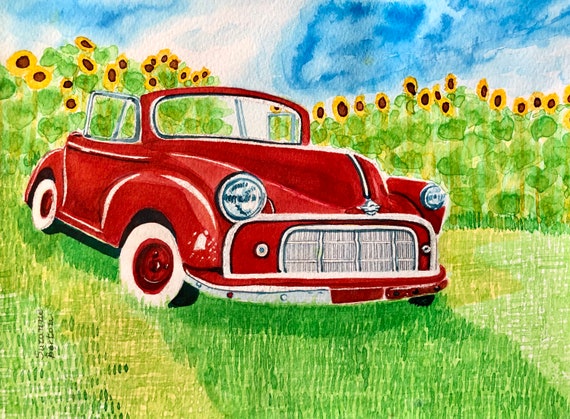This vibrant painting depicts a vintage red convertible car, likely from the 1940s or 1950s, with a characteristic rounded design and abundant chrome detailing. The car, parked in a field of meticulously painted green grass, features large white-wall tires with red hubs and prominent rounded headlights, one slightly smaller than the other, adding a whimsical touch to the scene. At the front, the car boasts a robust steel grill, partially chromed, with a mix of red and silver bumpers hinting at some wear and tear. The background is dominated by a towering field of sunflowers, their vivid yellow blossoms crowning long, blurred green stalks. Above, the sky is a dynamic mix of blue with streaks of white, rendered with wide, swirling brushstrokes that evoke a classic watercolor style. The scene is framed with an intimate, storybook charm, emphasized by the small, black-printed signature of the artist, possibly Suzette Porton or Borton, adding a personal touch to this nostalgic, simplistic artwork.